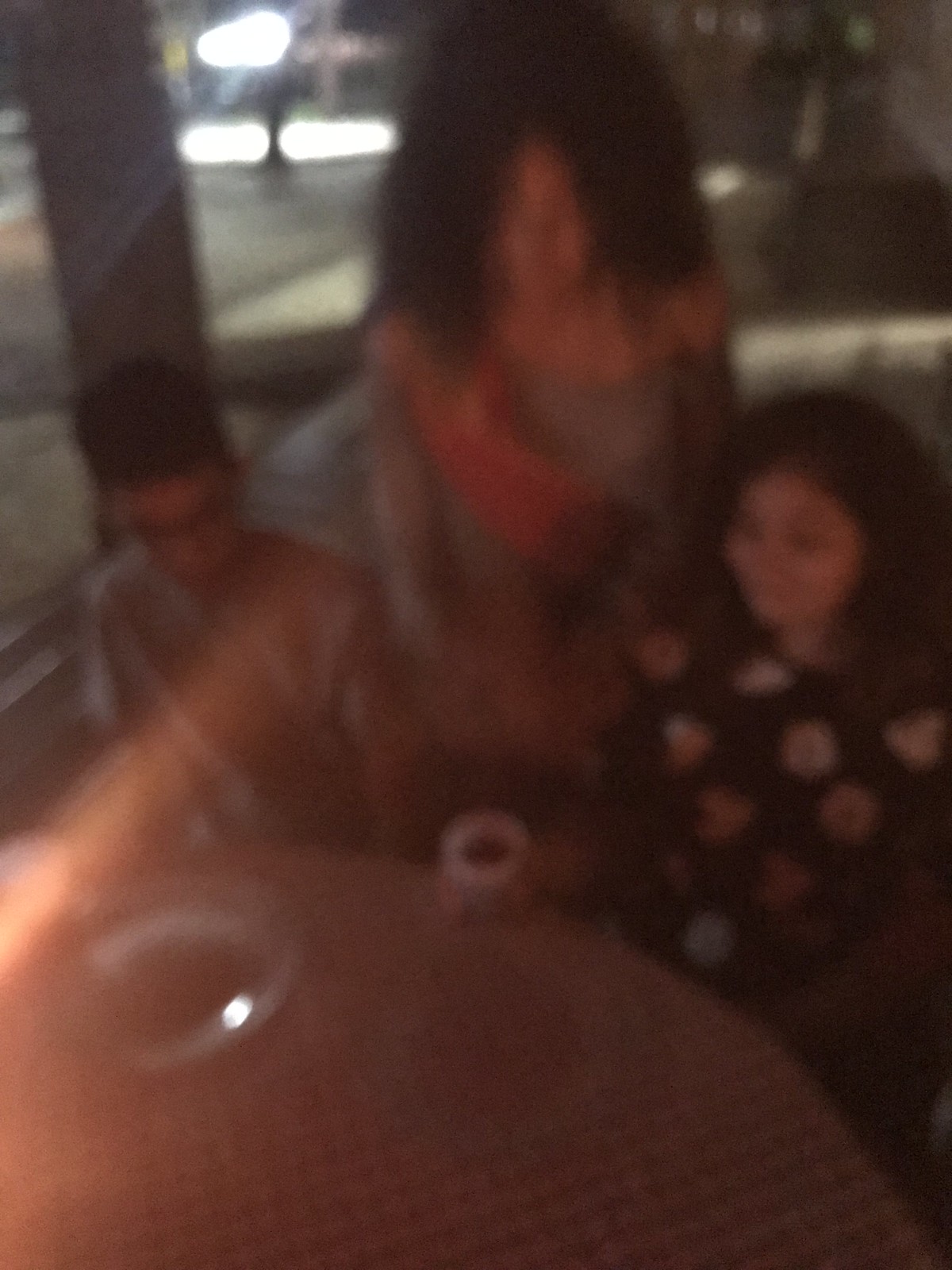A blurry, out-of-focus rectangular photograph captures a family scene with intricate details. The longer sides of the photograph are oriented horizontally. In the bottom left corner of the image, a round table adorned with a grey and white checkered tablecloth is visible. At the center of the table sits an empty, clear glass bowl. A light reflection stretches from the bottom right towards the top right corner, subtly illuminating the scene. 

Seated at the opposite end of the table is a young boy wearing black glasses and a short-sleeved grey shirt. To his right, a young girl is dressed in a black elbow-length shirt patterned with white circles, holding a white cup filled with brown liquid in her right hand. Positioned between the children is an older woman in a grey long-sleeved shirt, distinguished by a red sash draped from her shoulder across her torso. Despite the photograph's blurred quality, the familial bond and the nuanced details of their attire and surroundings create a vivid and intimate portrayal.